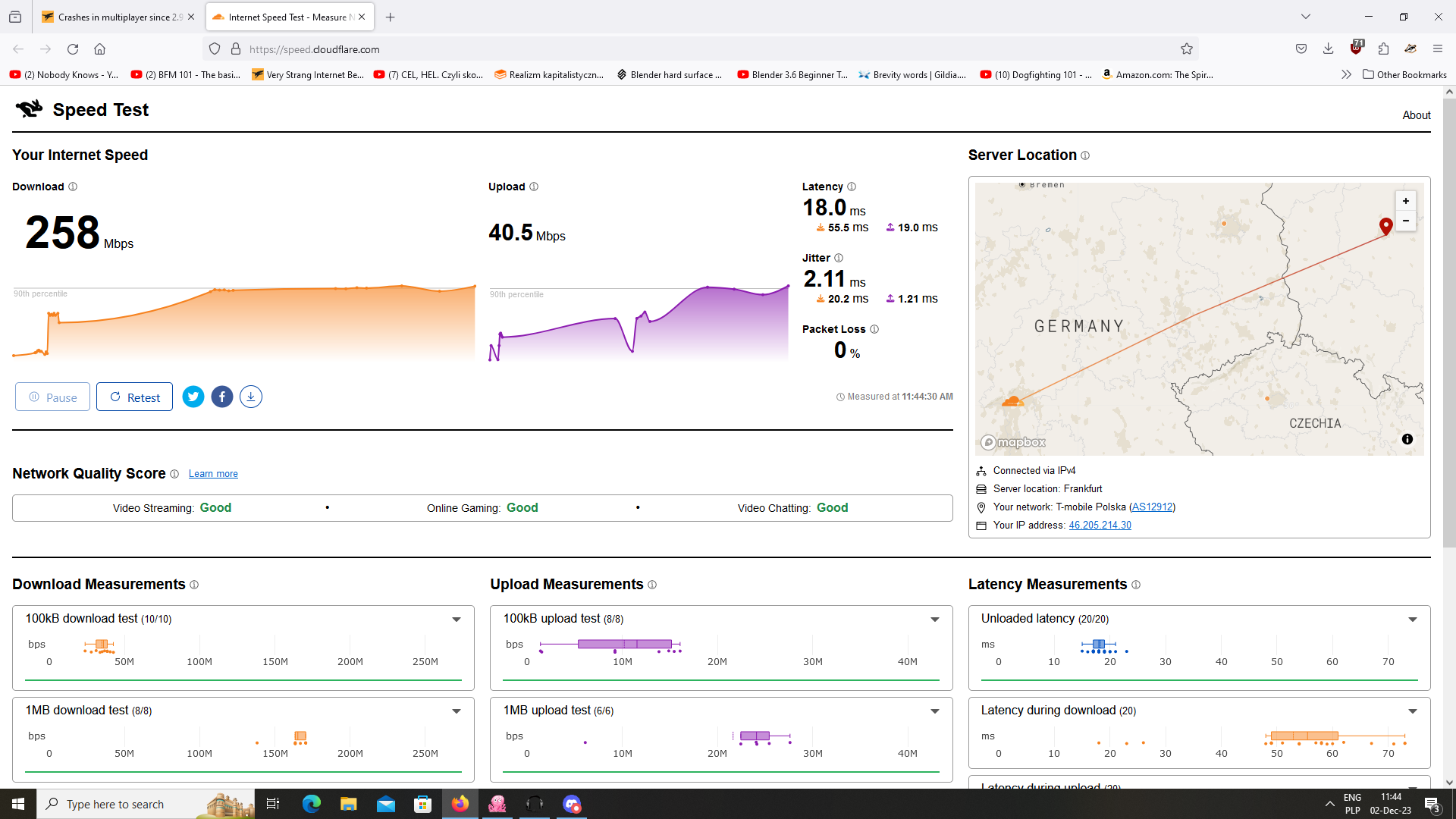The image depicts a web page designed for an internet speed test, prominently featuring a clean white background with primarily black text. Accentuating the monochrome are elements in purple, green, and orange-red hues. At the very top, the browser interface is visible, showcasing two tabs, with the active tab titled "Internet Speed Test."

Central to the web page, the title "Speed Test" appears in bold black letters accompanied by a rabbit icon. The speed test results are displayed below, indicating a download speed of 258 Mbps and an upload speed of 40.5 Mbps. Additionally, the results highlight a latency of 18 ms, jitter of 2.11 ms, and zero packet loss.

To the right side of the page, a map pinpoints the server location in Germany, specifically noting a connection to an IPv4 Frankfurt server via T-Mobile. The server's detailed address is "Pelowska."

At the bottom section of the page, a "Network Quality Score" is provided, evaluating the performance for various online activities: online gaming, voice chatting, and video chatting, all rated as "Good." Additional sections break down the measurements for download, upload, and latency, illustrated with respective graphs in orange and purple.

Overall, the image effectively captures a web page displaying a comprehensive internet speed test conducted on a browser, replete with detailed metrics and visual aids.